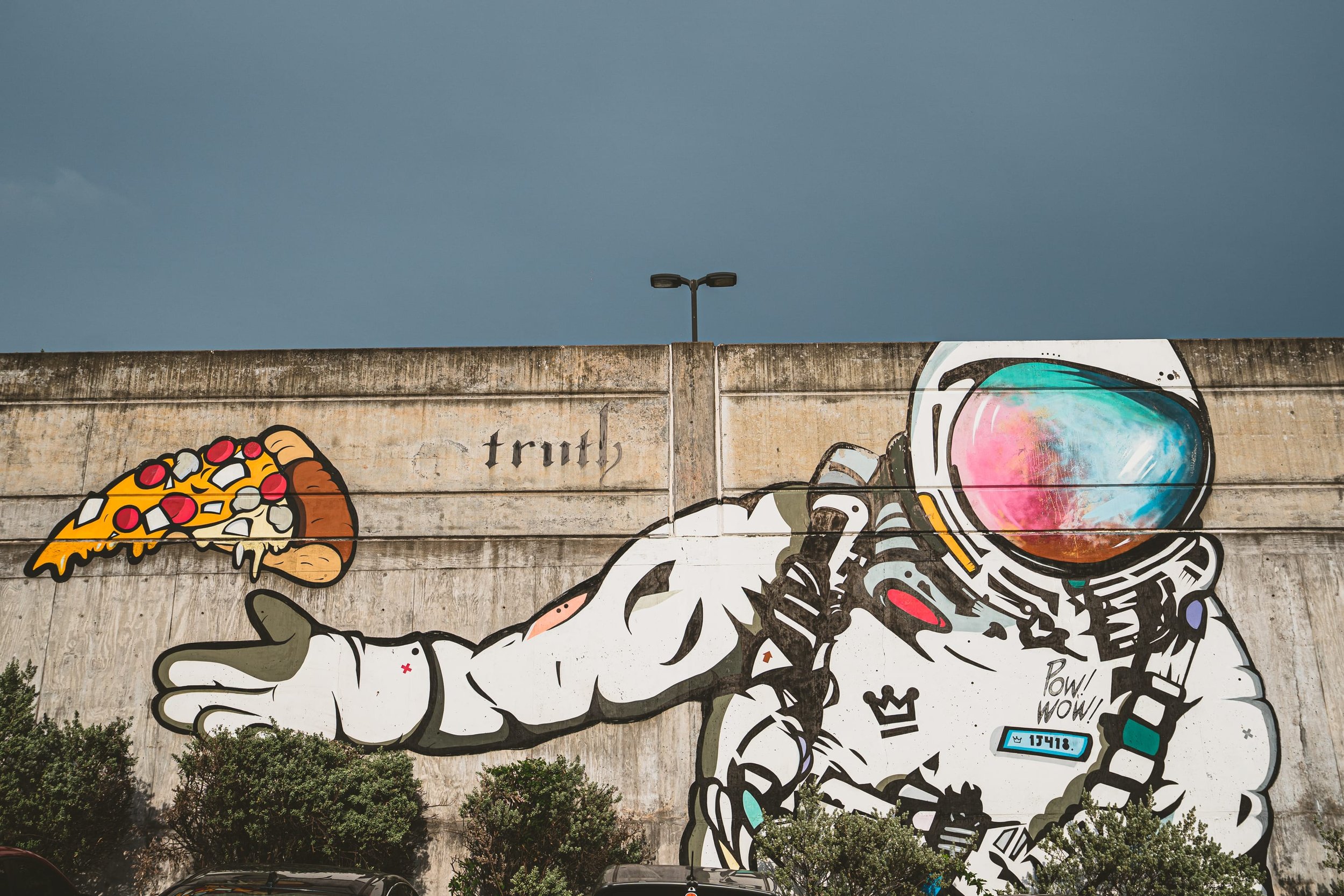This image is a detailed graffiti mural painted on an overpass or parking lot structure, featuring a vividly illustrated astronaut. The astronaut is wearing a full white spacesuit, including white gloves with a touch of green. The helmet of the suit exhibits an opalescent glow with hues of light teal, blue, and pink reflecting off of it. There is bold, black text on the front of the spacesuit that reads "POW WOW." In the astronaut’s extended right hand hovers a slice of pizza adorned with yellow cheese, red pepperoni, white onions, and mushrooms, creating the illusion that it’s floating in space. Above the astronaut's right shoulder, the word "TRUTH" is inscribed in a stylized font. The surrounding environment in the image includes a tree-lined horizon under a dark gray, overcast sky, hinting at impending rain. The mural is captured in a horizontal, rectangular photograph with an emphasis on the vibrant and fantastical elements of the astronaut and the floating pizza slice.